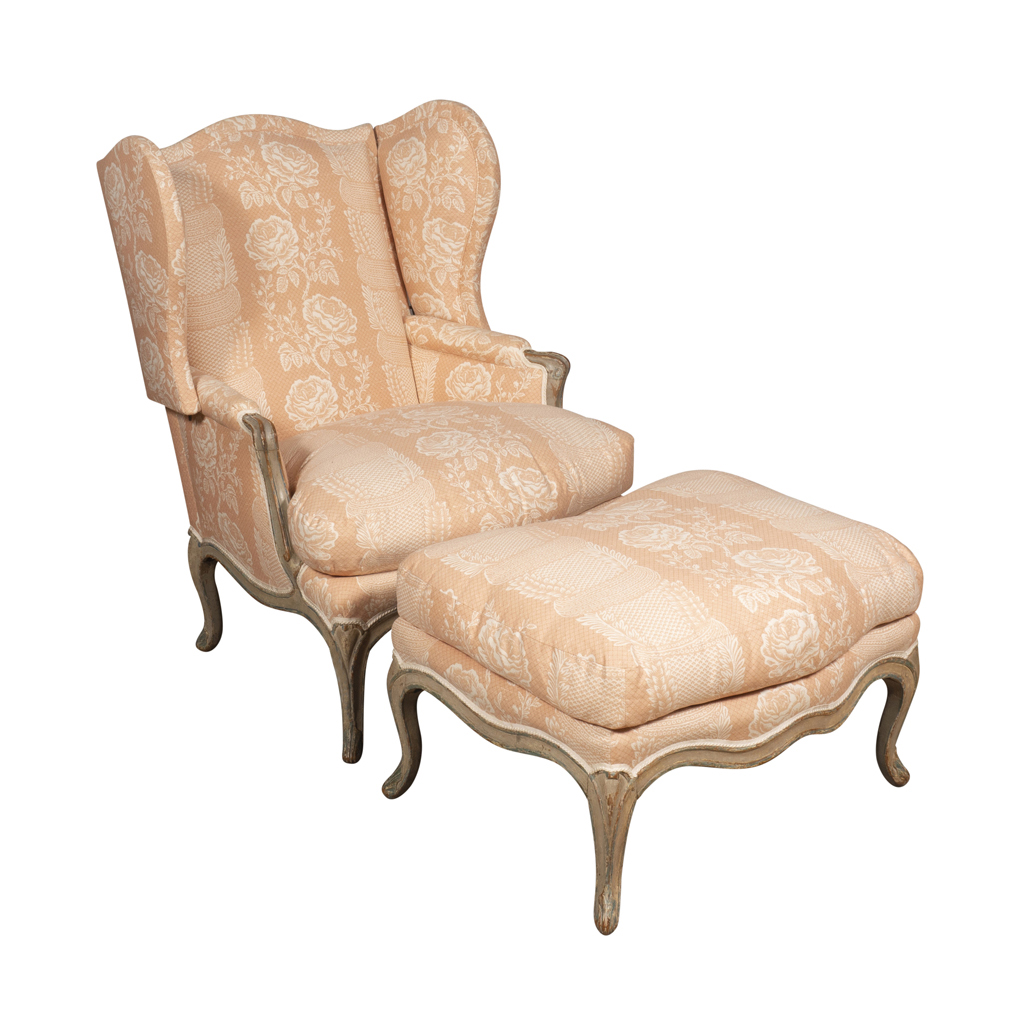This image depicts a finely crafted armchair accompanied by a matching ottoman, both designed to suggest a sense of elegance and comfort. The chair, with its high back and narrow armrests, is upholstered in a peach-orange fabric with a detailed white floral pattern. A distinctive wide pink stripe, adorned with a repeating white floral design, runs down the center of the chair's back and seat, continuing seamlessly onto the ottoman, creating a unified aesthetic. The chair features decorative, curved wooden legs, artistically shaped and brown in color, adding a touch of traditional charm. On each side of the chair are upholstered "wings" that match its fabric and design, providing additional support for resting one's head. The ottoman, separate yet complementary, mirrors the chair's upholstery and design, down to the intricately shaped wooden legs. The overall effect is both visually appealing and functional, inviting relaxation in a stylish setting.